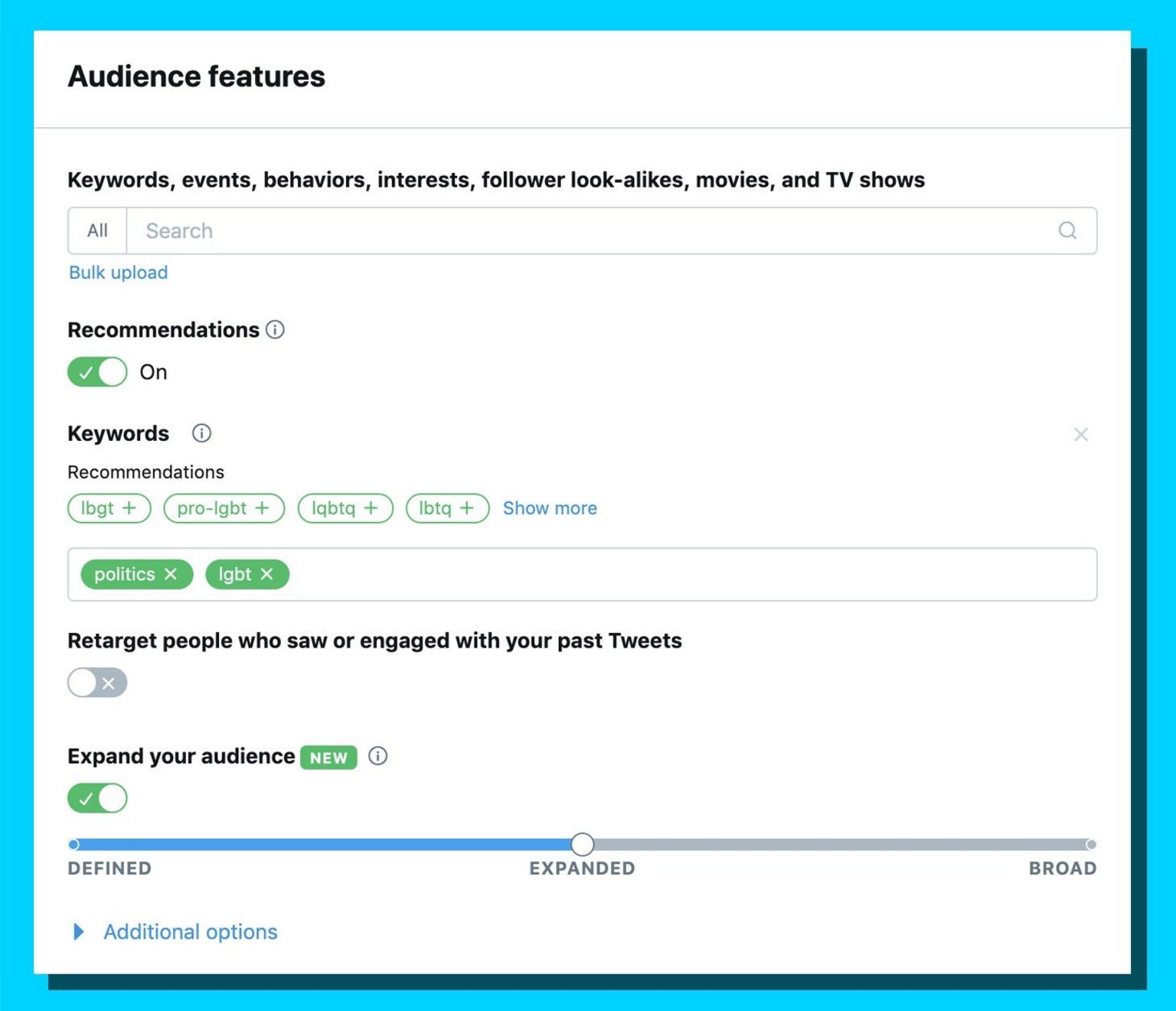This image is a screenshot from the settings or menu options section of an app that appears to be related to Twitter. The interface is framed by a bright, light blue border, resembling a picture frame, and features a mostly white background for the main content area.

At the top of the white background, the title "Audience Features" is prominently displayed in black text. Beneath this title, there is a long, rectangular white search bar for user input. 

Below the search bar, the first section titled "Recommendations" contains a toggle switch. The switch is currently toggled on, indicated by its green color with a white check mark.

Further down, the "Keywords" section features another bar similar in design to the search bar above, intended for entering keywords that the user prefers to receive more material about.

Next, the section titled "Retarget People Who Saw or Engaged with Your Past Tweets" has another toggle switch, which is toggled off in this screenshot.

The final section, labeled "Expand Your Audience," is marked with a "NEW" indicator in a green box. This feature is also toggled on. Beneath this, there is a slider bar with three options: "Defined," "Expanded," and "Broad." The slider is currently set to the middle option, "Expanded."